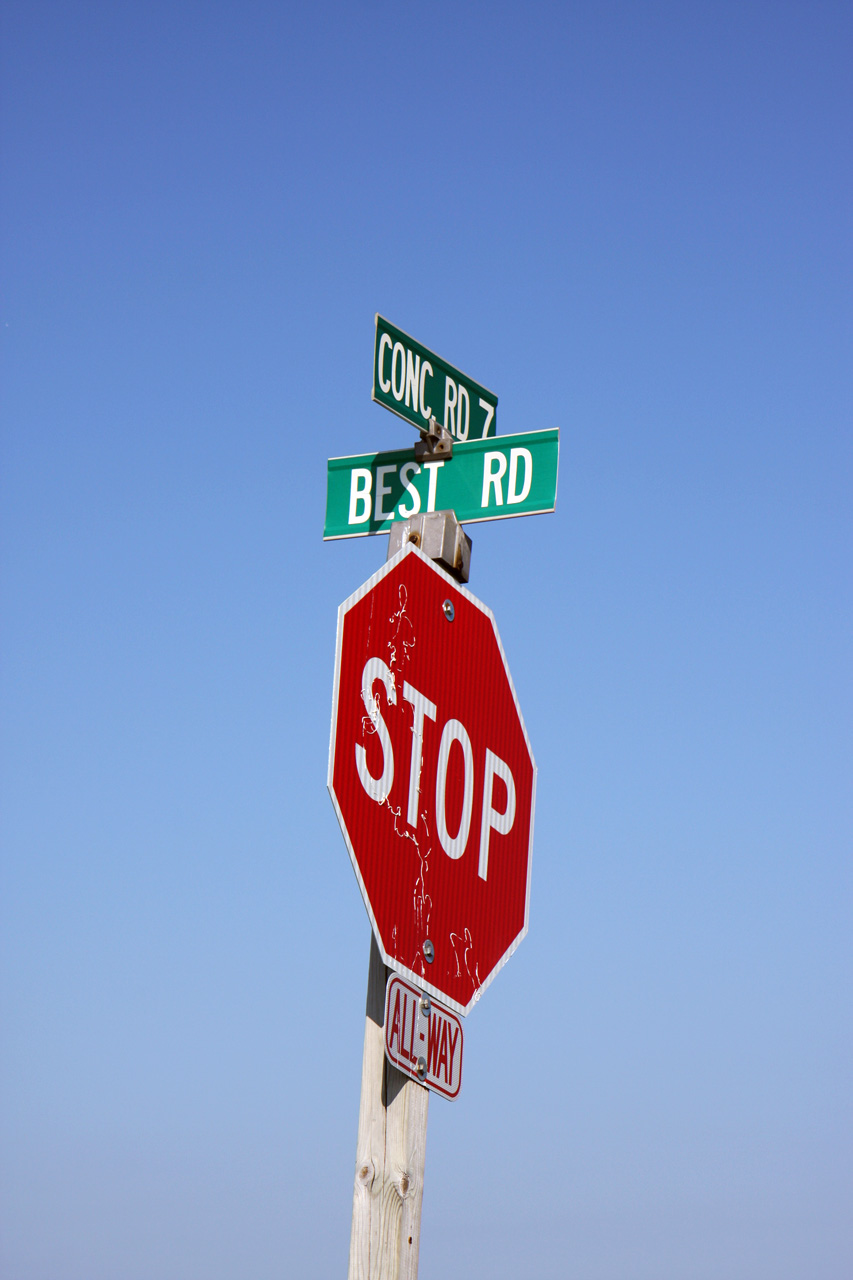The image captures a series of road signs mounted on a light gray wooden post. At the top, there are two green street signs — the uppermost reads "CONC RD 7" and directly beneath it is "BEST RD." Both street signs are green with white lettering. Below these street signs is a classic red and white stop sign, which is noticeably aged with white paint fading from the top left to the bottom right. Fastened below the stop sign, there is a rectangular red and white sign indicating "ALL-WAY" in capital letters, with a dash between the words. The signs are shot from a low angle, giving a clear perspective of the sky in the background, which graduates from a light blue at the bottom to a darker blue at the top. The photo captures the signs arranged in a T-formation, with the stop sign and "ALL-WAY" sign facing forward, while "CONC RD 7" and "BEST RD" face different directions.